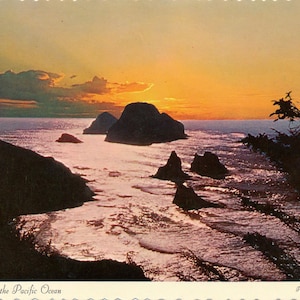This is a vintage square-shaped photograph capturing a stunning sunset over the Pacific Ocean, likely taken along the rocky coastline of northern California. The focal point is a serene cove with rock formations jutting out of the water, their dark silhouettes contrasting against the vibrant sunset. The sky exhibits a gradient of colors from deep orange near the horizon to light gray at the top, highlighting some clouds on the left side of the image. The ocean itself reflects a mesmerizing blend of purplish, blue, and silver hues due to the refracting light. To the left, the rocky cliffs meet the water, creating dramatic silhouettes, while a tree with branches and leaves intrudes from the right side of the frame, adding a touch of nature to the scene. At the bottom, a narrow white banner runs across with the words "The Pacific Ocean" written in the bottom left-hand corner, just above an incline of land featuring the silhouettes of bushes.